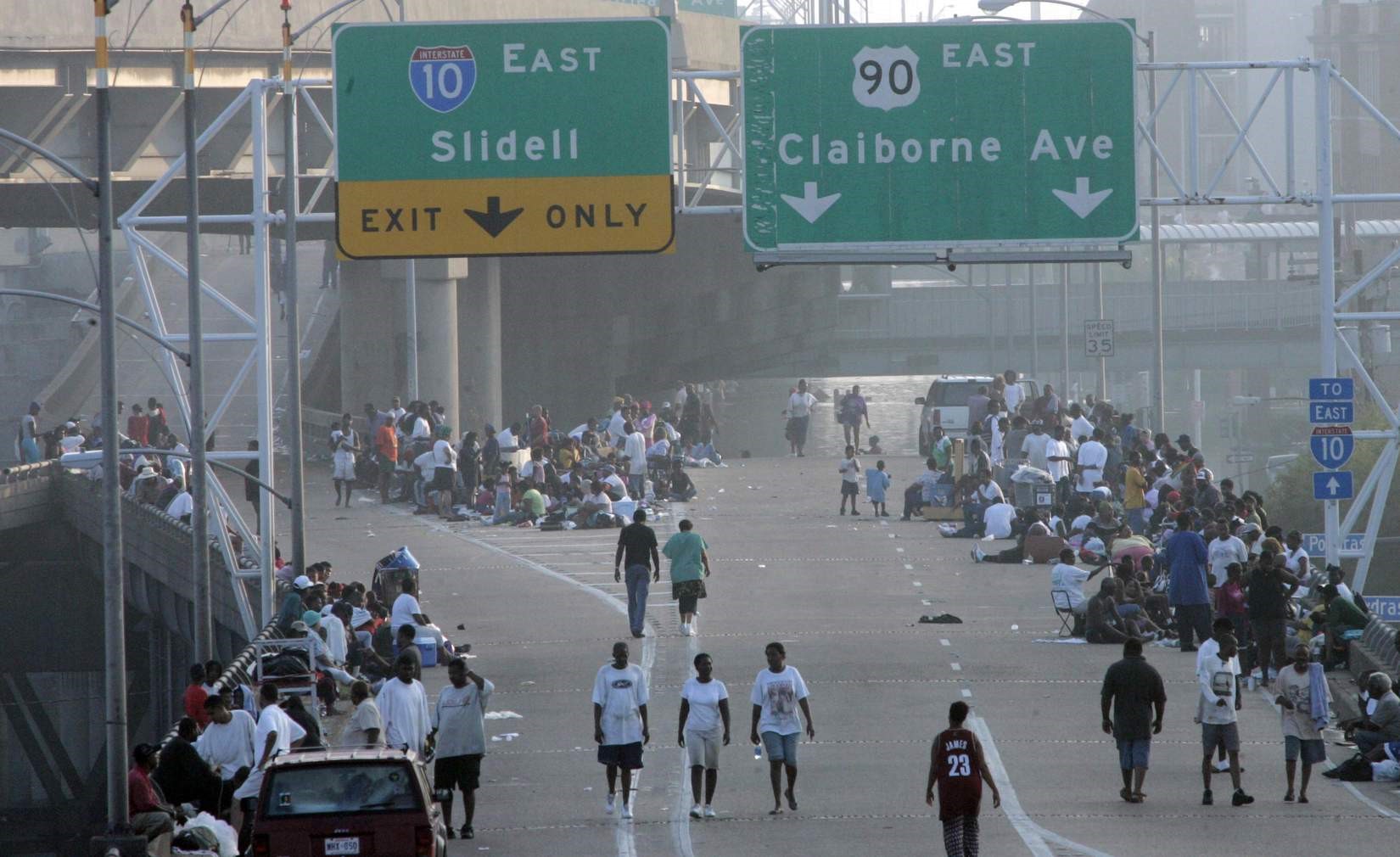This horizontally aligned rectangular image captures a highway overtaken by people participating in what appears to be a Black Lives Matter demonstration. Instead of vehicles, a multitude of individuals stands, walks, and sits along the roadway, halting traffic entirely. The scene occurs atop a bridge, where two highway signs can be seen overhead. The sign on the left signifies Interstate 10 East towards Slidell, accompanied by an "Exits Only" directive marked by a down arrow on a road construction orange or yellow background. The adjacent sign indicates Highway 90 East towards Claiborne Avenue, featuring two down arrows.

The highway, generally consisting of two lanes, diverges into a third for an exit on the left. A distinct dotted white line separates the lanes. Participants line the edges and median of the bridge, some seated and others standing, creating a vivid scene of human presence and unity. In the foreground, a few individuals in white T-shirts walk towards the camera. Two vehicles, presumably part of the demonstration, are also visible: an SUV parked in the bottom left-hand corner and another vehicle, possibly an SUV or pickup truck, visible in the distance. The collective occupation of the highway underscores the demonstrators' intent to disrupt normal traffic flow, marking their presence in a notable and peaceful way.